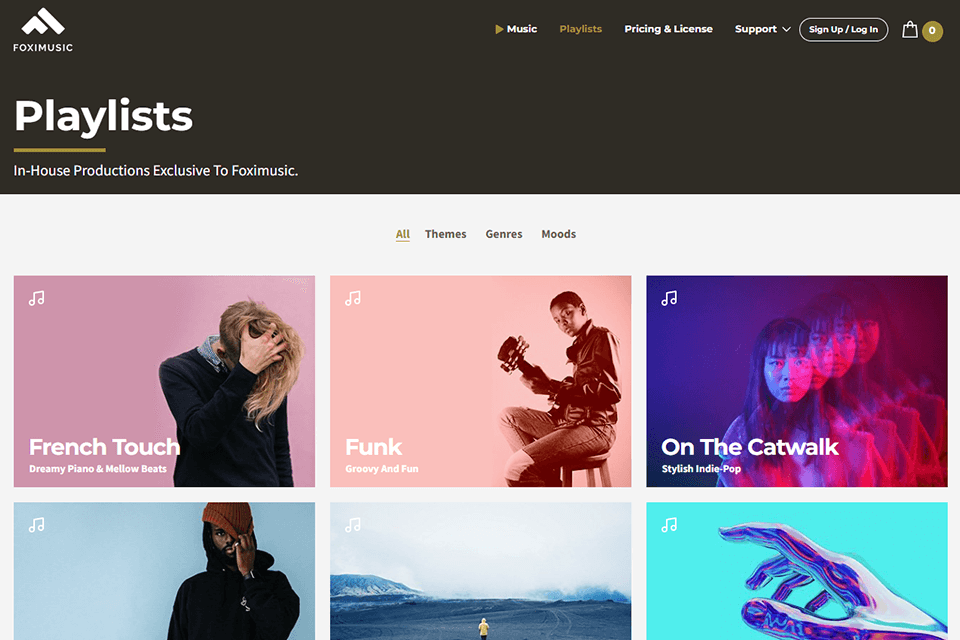In the given image, the focal element is a screen displaying a music service interface. At the very top of the screen, there is a large black rectangle featuring white text. On the top left corner of this rectangle, there is a stylized icon with an 'F', tilted sideways, followed by the label "Foxy Music" spelled out as F-O-X-I Music.

On the top right corner of the black rectangle, there are several navigation buttons labeled "Music," "Playlist," "Pricing and License," "Support," and "Sign Up/Log In." Adjacent to these buttons is a small shopping cart icon inside an army green circle, with a zero displayed, indicating an empty cart.

Beneath this header, a large white text reads "Playlist" accompanied by the subtext "In-House Productions Exclusive to Foxy Music." Directly below this, a gray navigation bar offers filter options labeled "All," "Themes," "Genre," and "Moods."

Under the gray bar, the main content area displays six distinct rectangular boxes, each featuring different images and textual descriptions.

1. The first box, located in the top left, has a pink background. It depicts a man wearing a sweater with long hair partially covering his face, and his hand resting on his head as he looks downward. The box is captioned with white text: "French Touch, Dreamy Piano and Mellow Beats."

2. The second box to the right features a peach background with an image of a person playing a guitar while seated on a chair and dressed in blue jeans. The text in this box reads: "Funk, Groovy and Fun."

3. The third box, characterized by bright colors including purple, pink, and blue, showcases a woman standing and facing forward. The image contains multiple overlapping shadows of the woman, creating a layered effect. The caption reads: "On The Catwalk, Stylish Indie Pop."

4. The fourth box displays a man with a light blue background. He is wearing a black hoodie and pulling down a wool cap over his head.

5. The fifth box has a scenic landscape featuring a person standing in the middle, wearing a yellow rain jacket.

6. The sixth and final box incorporates a turquoise and bluish-green color background with an image of a hand. The hand is uniquely colored like an oil spill with vibrant hues of neon blue, yellow, pink, and orange.

This detailed visual description encompasses the layout and content of the image, reflecting the elements displayed on the screen of the Foxy Music service interface.